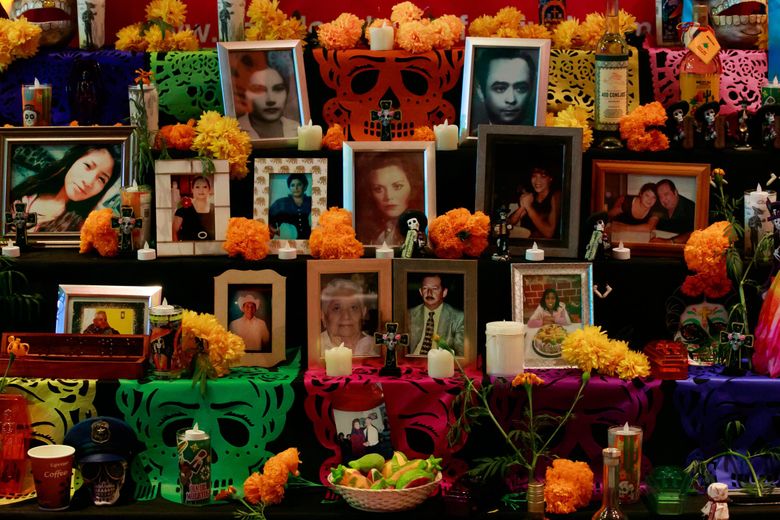The image depicts a vibrant, multi-level Day of the Dead altar, adorned with an array of colorful elements that celebrate the lives of the departed. Each shelf, draped with black blankets featuring ornate skull designs, is decorated with framed photographs of people of various ages, including a couple situated on the top right. These photos are surrounded by abundant bunches of bright orange marigold flowers, traditionally used in Day of the Dead celebrations.

At the center of the top tier, a prominent cross with a skull in the middle commands attention, while scattered throughout the altar are votive candles, both real and battery-operated, contributing a warm and reverent glow. Distinctive Mexican-style skeletons, painted in vibrant hues of blue, red, purple, and yellow, hang from the shelves, adding a touch of whimsical reverence to the scene. Additionally, the altar is dotted with small, decorated skulls, including one notably wearing a captain's hat.

Below the photos, on the lowest tier, a bowl of dragon fruit and other foods, a bottle of alcohol, and a red cup are placed in a basket, symbolizing offerings for the deceased. The overall setup, rising like stair steps, is meticulously arranged with each level showcasing a blend of floral arrangements, candles, and meaningful mementos that capture the essence of the Day of the Dead.